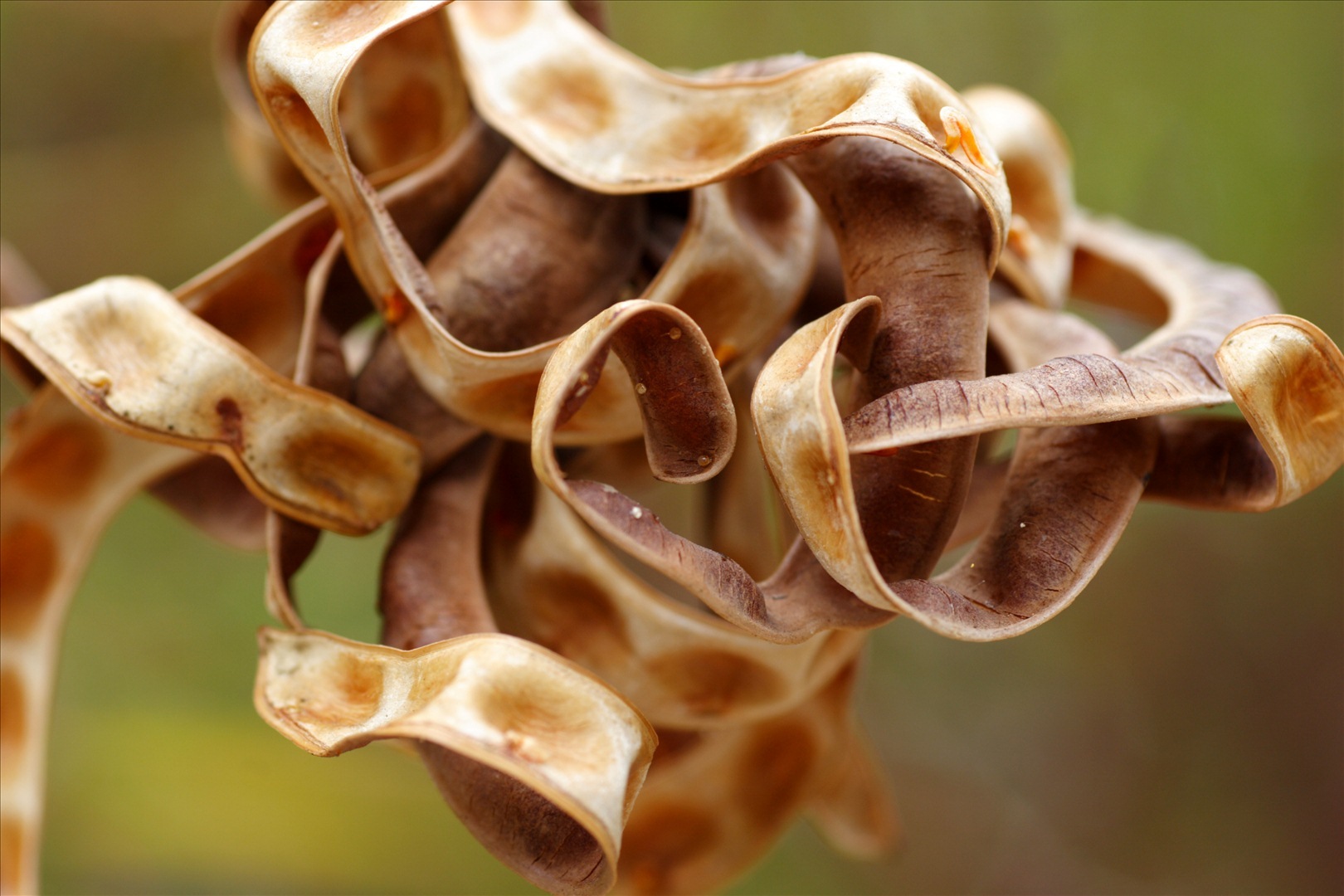This photograph, taken outdoors during the daytime, captures a detailed close-up of a long, dried brown seed pod. The seed pod is intricately curled and tangled upon itself, measuring approximately four inches when stretched and about half an inch in width. Its outer skin is a dark, burnt brown, while the inner side reveals a white or cream color adorned with light brown and gold patches, indicating where seeds once resided. The blurred background displays a gradient of colors, with the upper left corner showing a brownish-green hue, shifting to a greenish tint on the upper right, and transitioning to a yellowish-green in the lower left, with the lower right corner returning to a brownish tone. The photograph, rectangular and about six inches wide by four inches high, highlights the exquisite details of the seed pod against the softly blended, muted hues of the background.